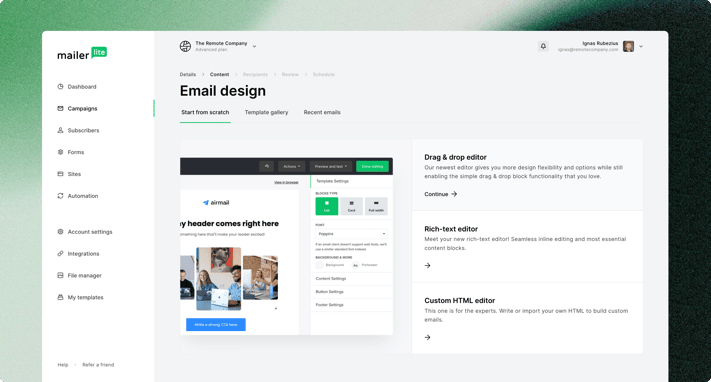The screenshot depicts a webpage from the MailerLite website, set against a green background with darker side panels on both left and right halves. The MailerLite logo is prominently displayed in the top left corner, with "Mailer" in white and "Lite" in green.

The left sidebar features the main navigation menu, which includes options like Dashboard, Campaigns, Subscribers, Forms, Stats, Sites, Automation, Account Settings, Integration, File Manager, and My Template. The currently open page is "Campaigns," indicating that the user is in the process of creating or managing an email campaign. The header of this section indicates that the email design was created by "The Remote Company."

Within the Campaigns section, various tabs are visible such as Start From Scratch, Templates, Gallery, and Recent Images, with the "Start From Scratch" tab highlighted. The content area features an interface for creating an email campaign with options like Drag and Drop Editor, Rich Text Editor, and Custom HTML Editor listed on the right side of the page.

The layout includes a black header area and several interactive buttons: a blue button at the bottom and a green button at the top right corner. At the top right of the page, there is a user profile section, showing a blurry profile icon, username, and profile picture, indicating that the user is logged in but the specific details are not clear.